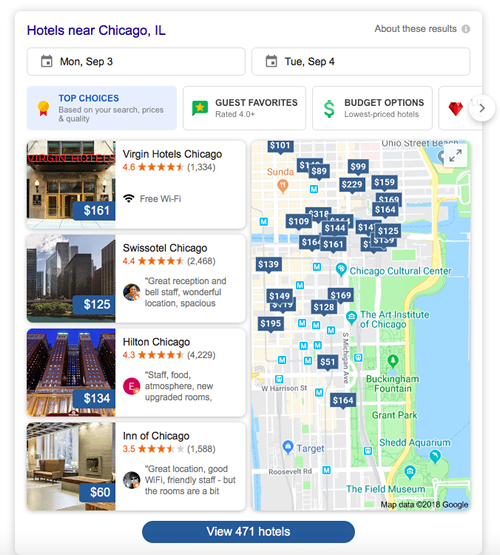**Detailed Caption:**

This image is a detailed screenshot likely taken from a smartphone, tablet, or computer screen, displaying hotel options in Chicago, Illinois. The search criteria specify a stay from Monday, September 3rd to Tuesday, September 4th. 

On the left side of the screen, the top hotel choices are highlighted with icons indicating award-winning status. The first hotel listed is the Virgin Hotel Chicago, priced at $161 USD per night, offering free Wi-Fi, and rated 4.6 out of 5 stars.

Below the Virgin Hotel is the Swissôtel Chicago, costing $125 USD per night. It has been favorably reviewed for its reception and bell staff, wonderful location, and spacious rooms, earning a rating of 4.4 out of 5 stars.

The third option is the Hilton Chicago, charging $134 USD per night. This hotel has a 4.3 rating and reviews praise its staff, food, atmosphere, and newly upgraded rooms.

Next is the Inn of Chicago, priced at $60 USD per night, with a rating of 3.5 out of 5 stars based on approximately 1588 reviews. Feedback highlights its great location, good Wi-Fi, and friendly staff, although the rooms are noted to be somewhat small.

To the right of the screen, an interactive map displays blue icons indicating the locations and prices of various hotels. By clicking on these icons, users can access more detailed information about each hotel directly on their device.

This thorough view provides a range of hotel choices from luxury to budget-friendly options, allowing users to make an informed decision based on their preferences and budget. The overall search results are clearly laid out for a stay in Chicago, Illinois on the specified dates.